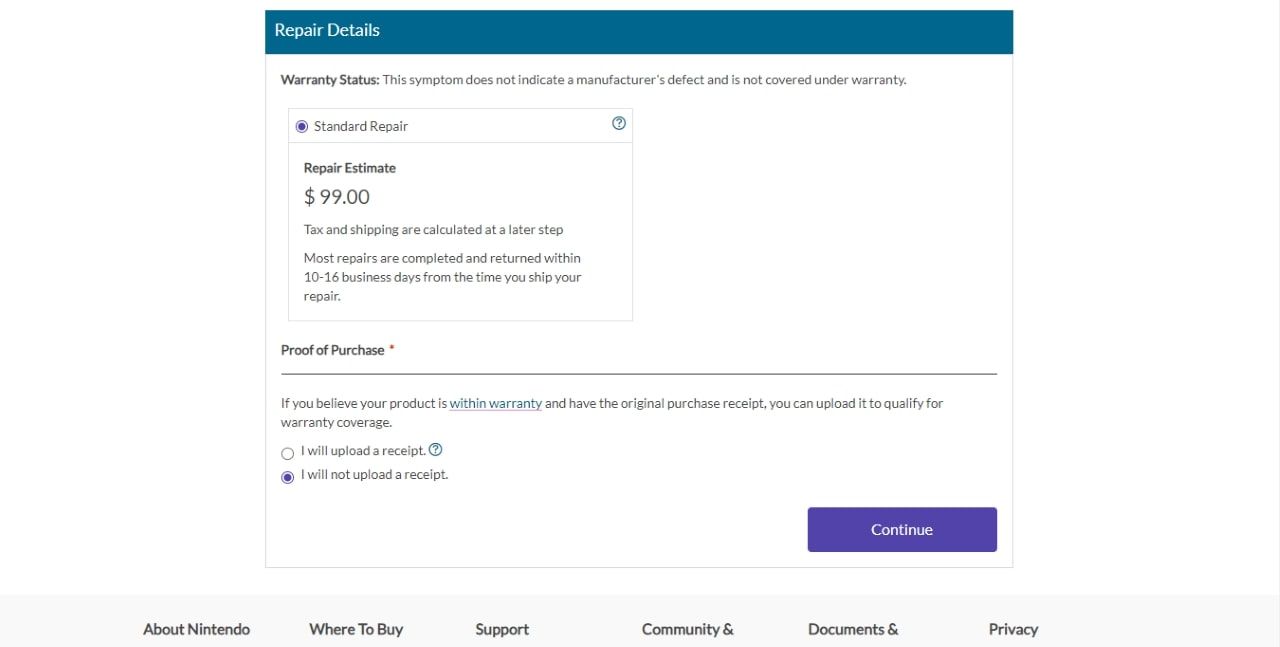The image depicts a webpage designed for detailing payment options and repair information, characterized by a professional, clean layout. At the top, a sky-blue banner prominently displays the title "Repair Details." Directly below, the term "Warranty Status" is bolded in black, signifying an important section. Positioned to the right of this heading, there's a notification stating, "This symptom does not indicate a manufacturer's defect and is not covered under warranty."

Beneath this notification, a rectangular box labeled "Standard Repair" is displayed, accompanied by a blue-filled circle. Adjacent to this, a circle containing a question mark offers additional information upon interaction. Following this section, the text "Repair Estimate" is prominently shown, including a specified amount of $99.00. A note explains that tax and shipping costs will be determined at a later step.

Further down, the phrase "Proof of Purchase" is highlighted, marked by an asterisk slightly above the 'E' in "Purchase". A horizontal black line separates this area from the subsequent text, which advises that users can upload their original purchase receipt to qualify for warranty coverage if they believe their product is within the warranty period.

Below this instruction, there are two radio buttons for user selection. The first option, "I will upload a receipt," is paired with a question mark in a circle, offering further clarification if needed. The second option, "I will not upload a receipt," is highlighted and selected by default, indicated by a filled-in circle.

At the bottom-right corner of the page, a blue rectangle button labeled "Continue" invites users to proceed to the next step.